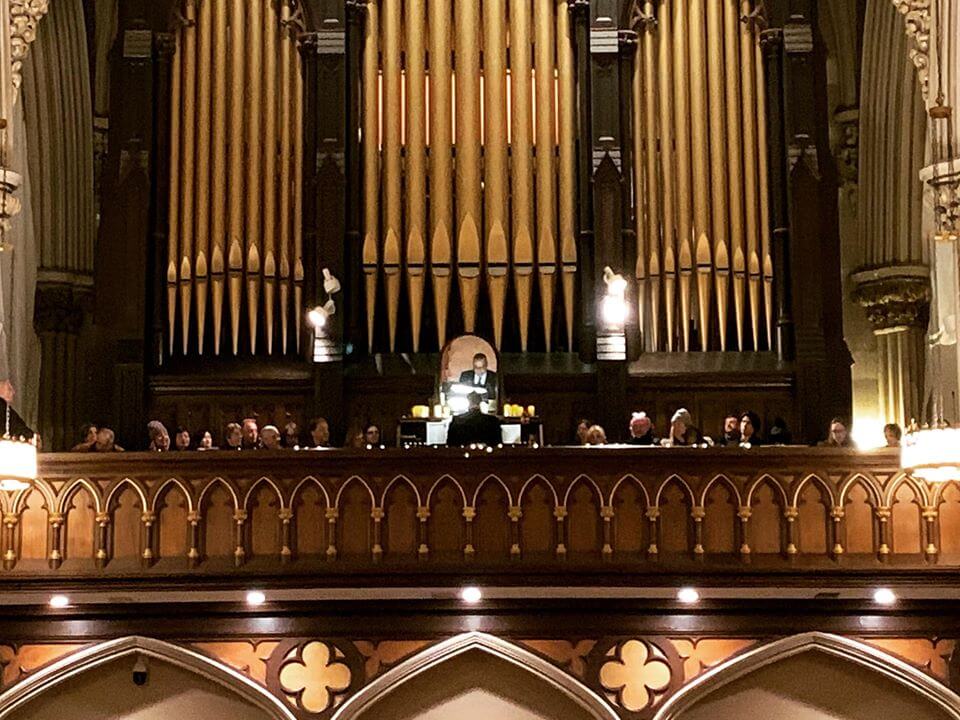This wide-angle indoor photo, likely taken in a cathedral or concert hall, captures a grand and detailed scene centered around an impressive large pipe organ with rows of golden pipes. Situated against the back wall, the organ is flanked on both sides by faintly illuminated statues, partially obscured by a flash of light. Below the organ, a wooden balcony with an arched facade extends across the image, adorned with intricate archways and floral-like decorations. 

Audience members are present on both the left and right sides of the balcony, and a man standing on a podium in the middle directs his attention towards the organ. Another man is seen emerging from a doorway directly beneath the organ. The balcony's design features recessed lighting with five round lights illuminating the space.

In front of the balcony, chandeliers hang from the ceiling at about the same height, their white and gold trim adding to the opulent ambiance. At the bottom of the photo, three arched doorways can be seen. Additionally, on the piano to the side, adorned with yellow candles, a pianist plays behind sheet music while a conductor in a white shirt, black tie, and black suit stands prominently. A large mirror is positioned in front of the organ player, possibly to allow spectators a view of his face. This gathering appears to be a blend of spectators and chorus members, contributing to a rich auditory and visual experience.